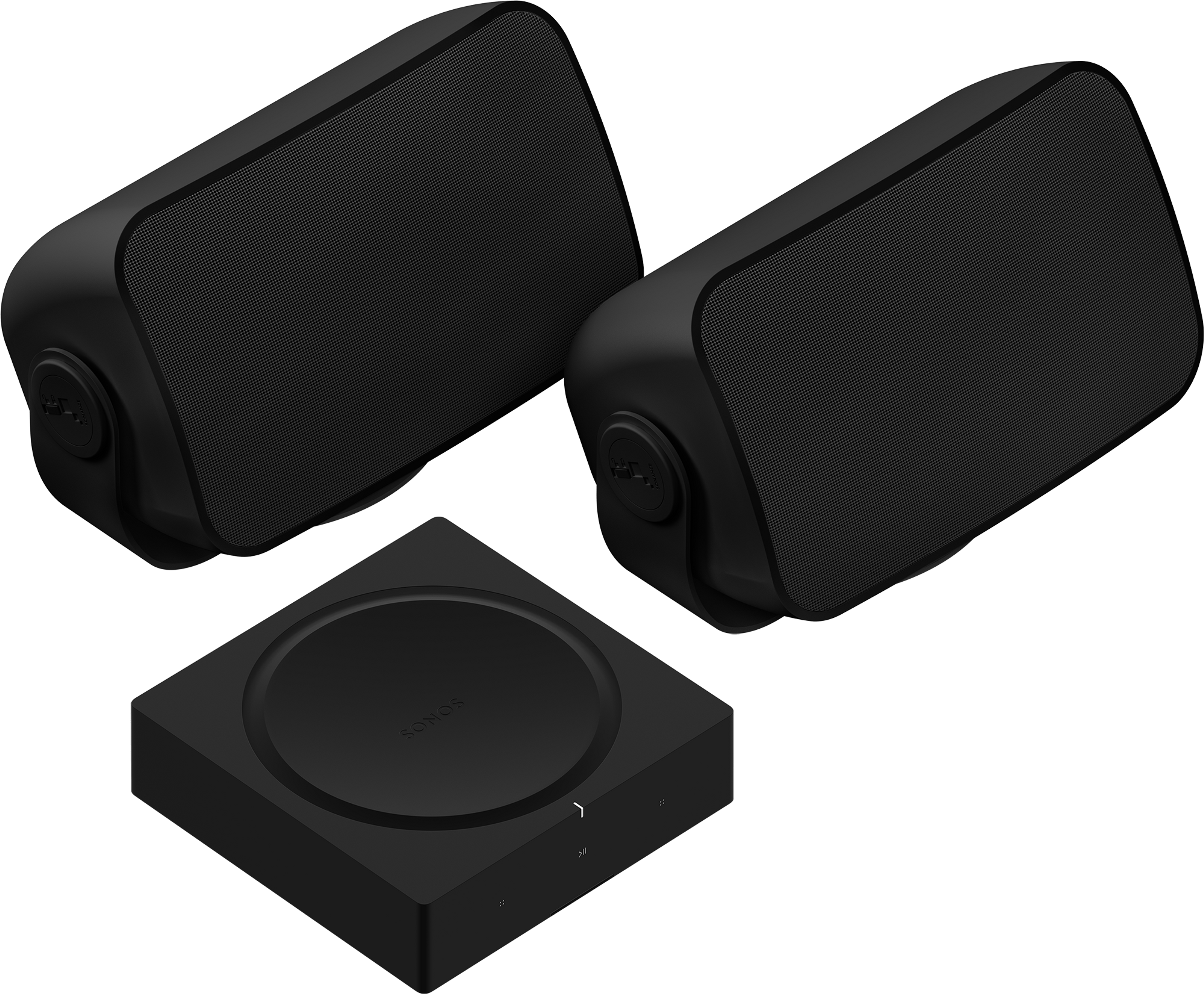This image features a product listing for a set of portable, black Bluetooth speakers. The main focus is on two rectangular speakers that are sleek and wireless, as there are no visible cords. These speakers are displayed at an angle, offering a view from the right side, and arranged one slightly in front of the other. Accompanying these speakers is a smaller, black, square object with a circular imprint in the middle—possibly a charging port or an accessory that complements the speakers. The entire setup appears to be professionally photographed on a white background, reminiscent of a typical Amazon product advertisement, suggesting a compact, portable design tailored for easy mobility.